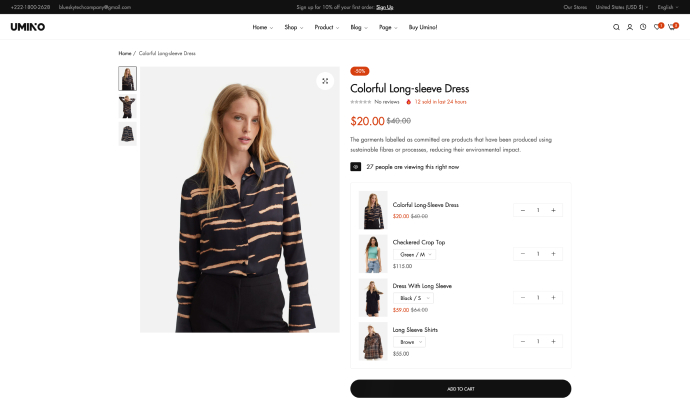The image showcases a vibrant and user-friendly web page for Yumino, an online shopping platform. The navigation menu at the top lists categories like Home, Shop, Product, Blog, and Page, providing easy access to different sections of the site. A banner promotes a special offer: "Sign up for 10% off your first order," encouraging user registration. 

Below the banner, there is information about Yumino's physical stores located in the United States and language options, currently set to English. 

A featured product is a colorful long sleeve dress, available for $20, marked down from $40. This dress is highlighted as part of their "committed" collection, meaning it is made from sustainable materials and processes that minimize environmental impact. The item has no reviews yet but has seen 12 sales in the past 24 hours.

The web page also showcases other fashion items. A checkered crop top is listed at $115 with a quantity of one available. A long sleeve shirt is priced at $55, with one in stock. Additionally, a dress with long sleeves is offered for $59, also with a quantity of one. 

Overall, the web page effectively combines product details with promotional content to attract and inform potential customers.